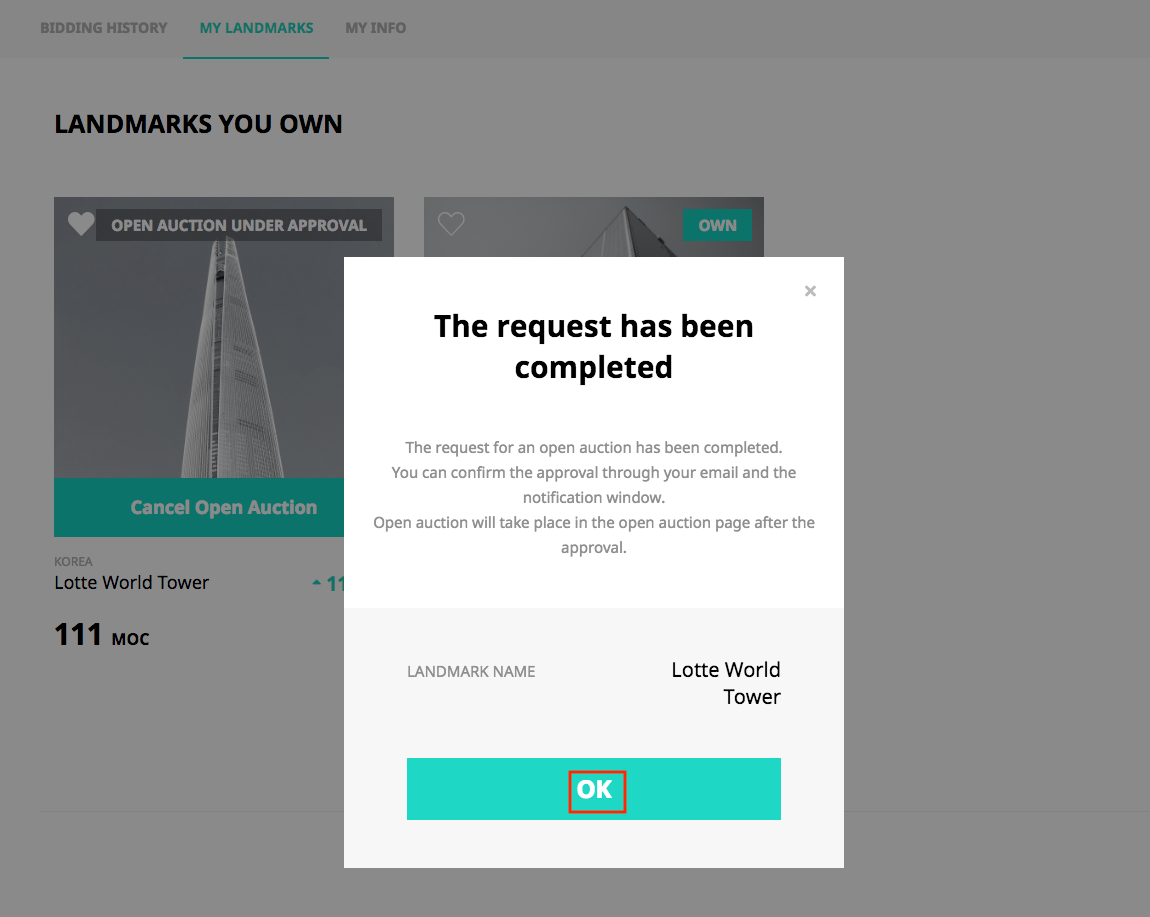The image displays a large, vertically aligned, square-shaped interface with a grayed-out background, overlaid by a prominent white pop-up box that requires user action. In the upper left-hand corner, the title "Bidding History" appears in gray. Below it, the tab labeled "My Landmarks" is highlighted in seafoam green and underlined, while "My Info" appears in gray. The section titled "Landmarks You Own" is in black, along with the option "Cancel Open Auction."

The partial image of a very tall building, identified as the Lotte World Tower in Korea, is visible but mostly obscured by the pop-up box. A heart icon is in the upper left corner of the image, indicating the option to favorite the landmark. The text next to the image reads: "Open Auction Under Approval, Korea, the Lotte World Tower, 111 MOC." 

Within the pop-up box, it states in black text: "The Request Has Been Completed." A gray "X" is in the upper right corner of the box for closing it. The message continues: "The Request for an Open Auction Has Been Completed. You can confirm the approval through your email and notification window. Open Auction will take place in the Open Auction page after the approval."

Towards the bottom of the box is a gray-background section labeled "Landmark Name" in black, followed by the text "Lotte World Tower." The box also contains a prominent "OK" button in seafoam green with white lettering, outlined by a red box.